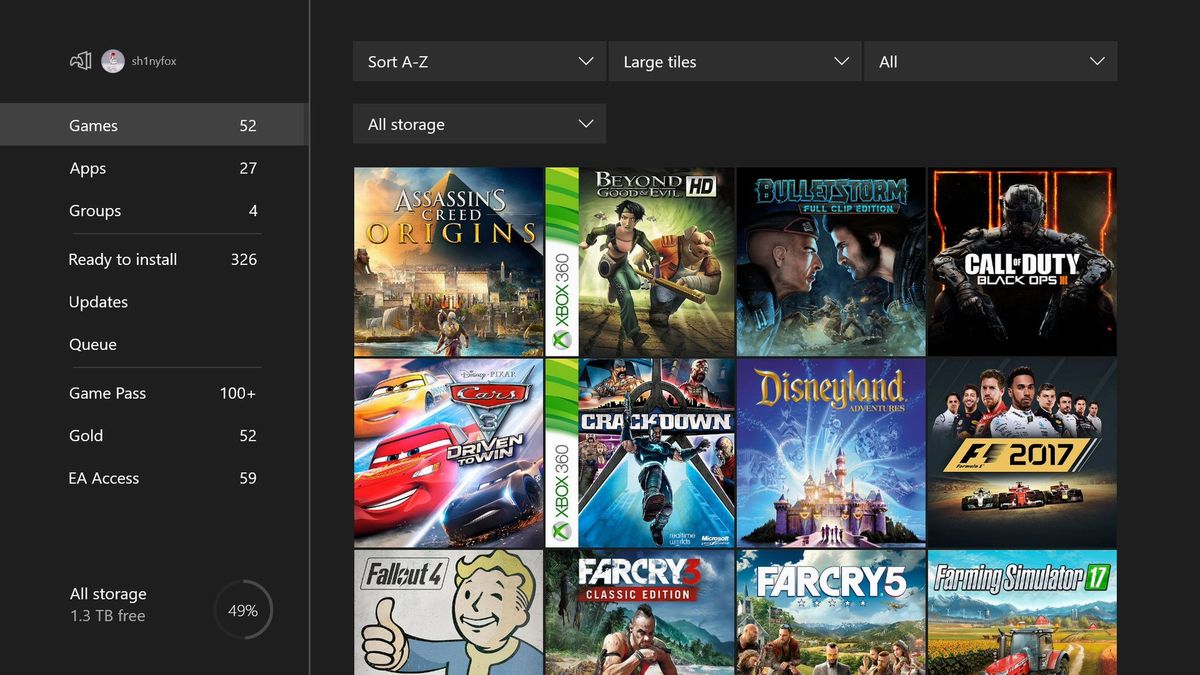The image showcases a comprehensive and organized digital library interface from a website dedicated to various games, Xbox 360 titles, and movies, all set against a sleek black background. To the left side, prominently displayed is a user profile named SH1NYFOX, represented by a white and gray avatar. Below this profile, detailed statistics are listed: Games (52), Apps (27), Groups (4), with additional categories including Ready to Install (326), Updates, and Quive. There's also specific information about subscription services: Game Pass (100+), Gold (52), and EA Access (59). 

Storage information is clearly presented, showing 1.3 TB free, which equates to 49% utilization, visually represented by a circle that is nearly half shaded gray. At the top of the interface, there are options for organizing the content, including Sort A to Z, Large Tiles, All, and All Storage. The main section features an array of game icons, including prominent titles like Assassin's Creed, Beyond: Two Souls, Bulletstorm, Call of Duty, Cars 3, Crackdown, Disneyland Adventures (2017), Fallout, Far Cry, and Farming Simulator, giving a snapshot of the user's diverse gaming collection.